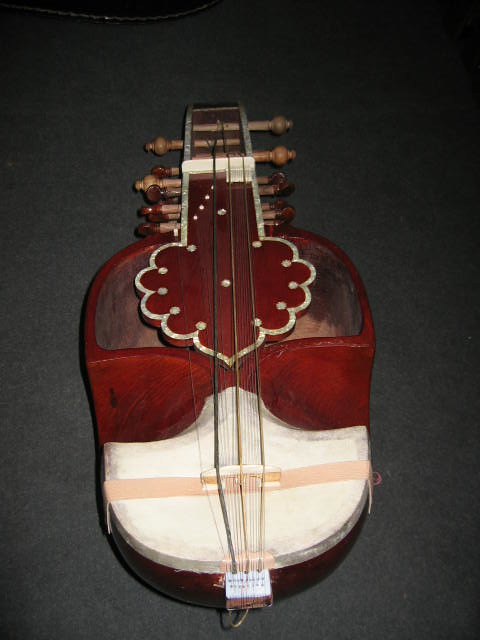This photograph showcases a unique and unfamiliar musical instrument, resembling a small guitar or possibly related to a ukulele. The setting is indoors, with a dark background and the instrument resting on a piece of cloth or carpet, suggesting the flash was used to capture the image. The instrument itself features a body that is partially red and partially white, with additional grayish panels. Its dimensions are smaller and more condensed compared to a typical guitar but larger than a ukulele, with a wider build. The strings, which vary in color from dark green to brown, and lighter green, stretch along the body. The top of the instrument, where the strings meet the neck, houses numerous tuning knobs, approximately eight on each side, crafted from light brown wood. This intricate and possibly old instrument, which could be on display in a museum, stands out against the black backdrop, highlighting its vibrant colors and detailed construction.